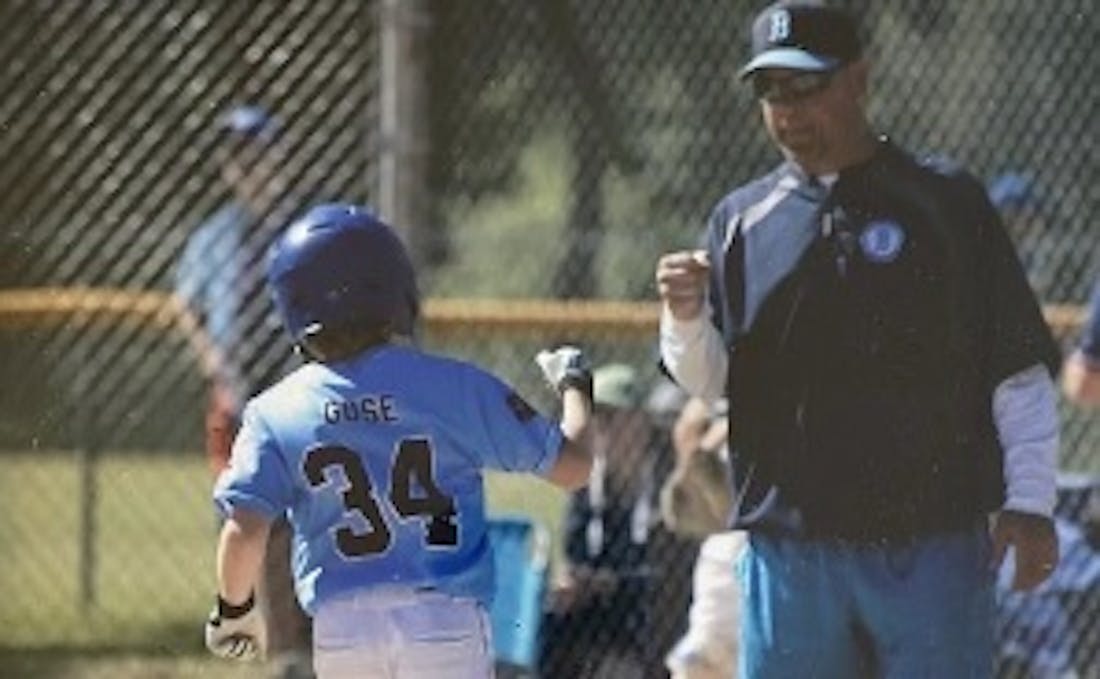The image captures a heartwarming moment at a little league baseball game, depicting a coach and a young player mid-celebration. The coach, facing the camera, is dressed in a blue hat with a bee emblem, matching sunglasses, a bee-logoed shirt layered over a white long-sleeved shirt, and blue pants. He extends his right hand, forming a fist, ready for a fist bump. The little boy, seen from the back, wears a blue helmet and blue jersey with the number 34 and the name "Guse." He’s also in white baseball pants and white gloves, mirroring the coach's gesture with his own fist raised. The background features a chain-link fence with a yellow top and blurred spectators, suggesting a lively game setting. Another individual in a blue shirt and hat stands near the fence, adding to the dynamic, supportive atmosphere of the scene.